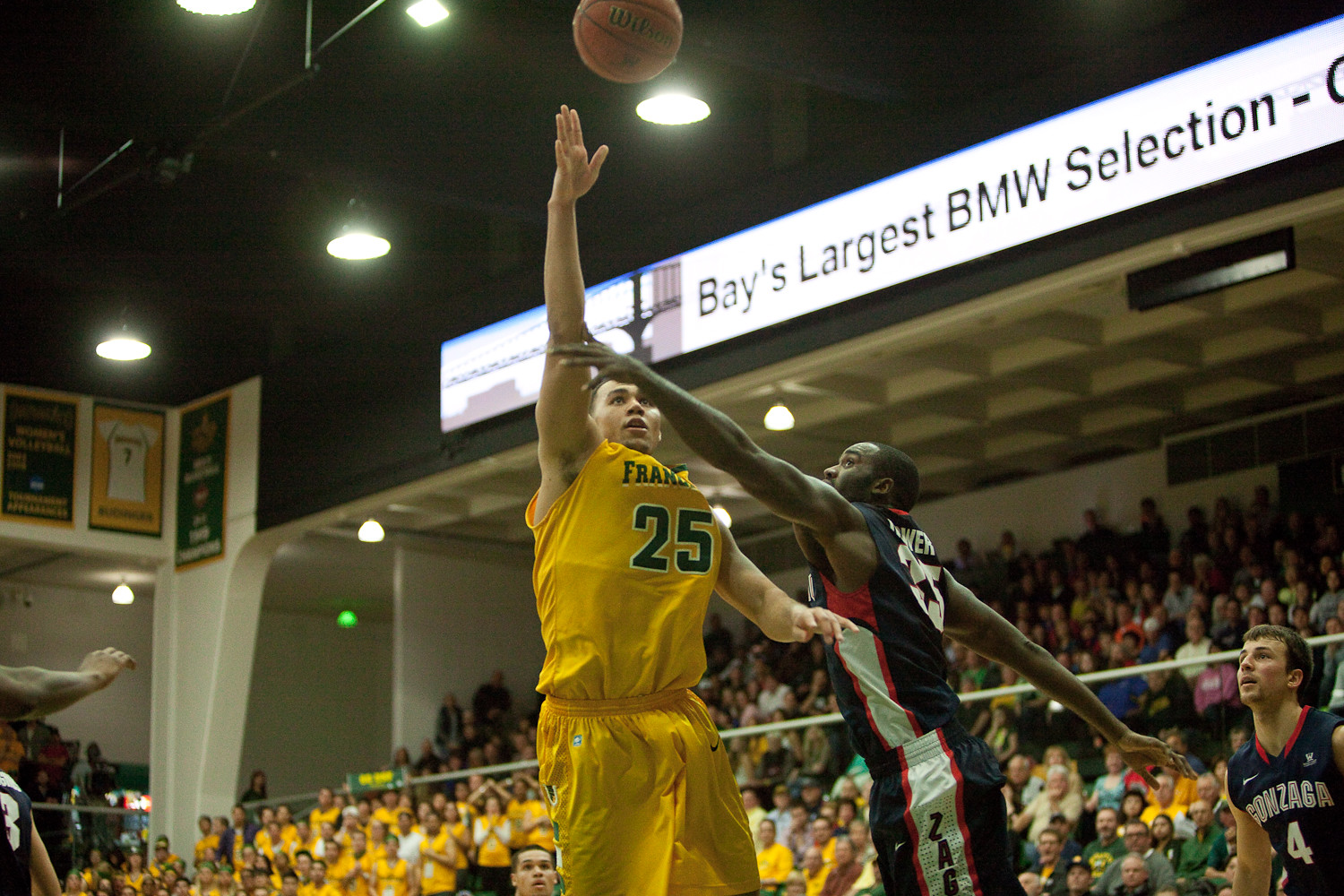The photograph captures a dynamic moment during a basketball game in a large gymnasium. High above the court, white lights hang from the beams, providing stark illumination against the dark ceiling, where a sign proclaims "Bay's largest BMW selection." The central focus features two basketball players in action: a white player in a yellow uniform with the number 25, seemingly taking a shot with his right hand elevated. The letters "F-R-A-N" are visible on his jersey, hinting it might spell "France." Opposing him is a black player in a red, white, and blue Gonzaga uniform, with a white stripe running down the side. This defender, wearing number 35, has his left arm outstretched in an attempt to block the shot. Another Gonzaga player, number 4, watches the action unfold, further back on the court. The scene is lively, with a large crowd situated on the right side, intently observing the game. In the foreground, only partial views of other players are visible, including just an arm and the right side of a back, adding to the sense of a crowded, tense moment in the game.